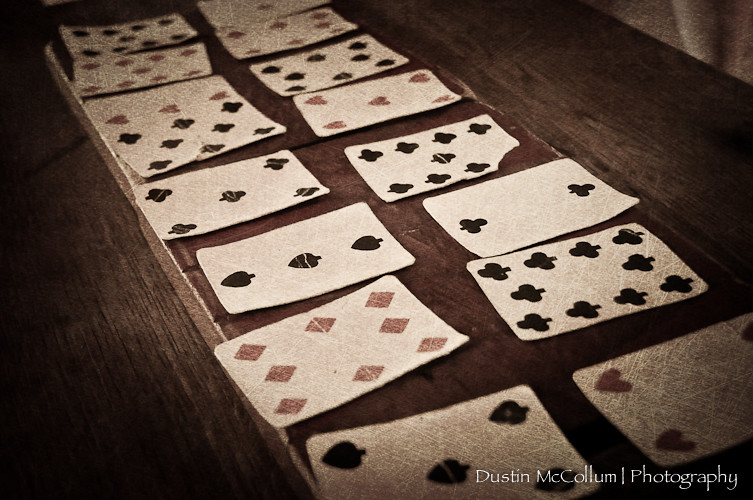This evocative photograph, tinted with a heavy yellow hue to create an antique, rustic aesthetic, captures a collection of vintage playing cards arranged in two rows of eight on a weathered brown wooden table. Viewed from a slightly off-center angle, the cards exhibit signs of age, with bent edges, corners, and visible scratches adding to their nostalgic charm. The cards display simple images of suits—hearts, clubs, spades, and diamonds—but notably, no numbers accompany the suit symbols. Among the worn cards, the nine of clubs stands out with a missing corner, situated roughly in the center of the array. The overall composition lacks any deliberate pattern, contributing to its raw, unpolished appeal. The photograph is subtly signed "Dustin McCollum Photography" in small white font in the bottom right corner, completing its vintage narrative.